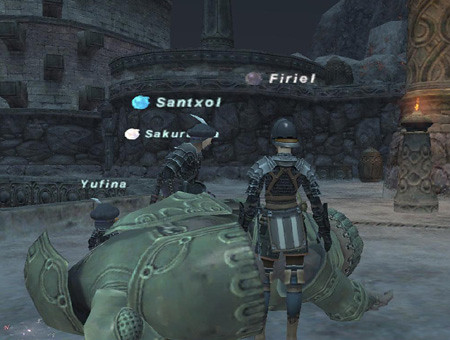In this gameplay capture, two soldier figures are prominently featured, each donned in a variety of armored shades including black, gray, silver, white, brown, and chocolate brown. Both are equipped with helmets, standing in proximity to a monstrous, turtle-like character. This creature is olive green with intricate carvings, though its face is not visible, and its legs can be subtly discerned.

Floating above the characters are various player or character names encased in differently colored circles. The name "F-I-R-I-E-L" is inside a brown circle, "S-A-N-T-X-O-L" appears in a blue circle, and "S-A-K-U-R" (with the last letter obscured) is within a super pale red circle.

The scene is set on a stone floor, with a dark, castle-like structure providing a historical ambiance in the background. Adding to the medieval atmosphere, there is a stone podium holding a visible flame, and stone carvings can be seen enhancing the castle's intricate detail.